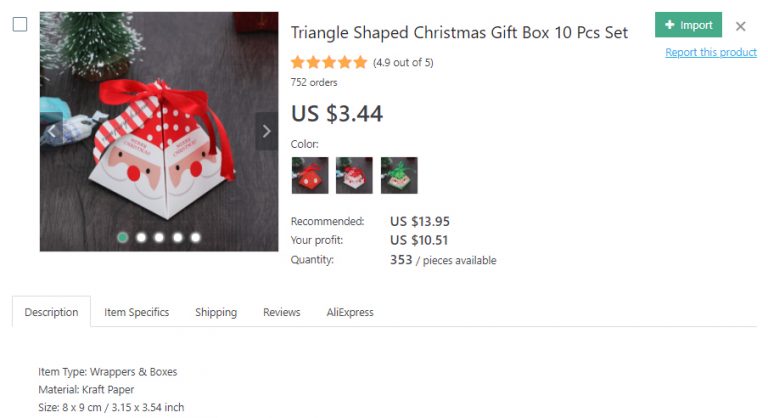The image is a screenshot of a product page, though the exact website or app is unclear. The top left of the image features a picture of the product, which is a triangular prism-shaped box adorned with Santa Claus faces on each side and topped with a red bow. The box appears to be sitting on a wooden floor. 

To the right of the image, the product title reads "Triangle Shaped Christmas Gift Box, 10-Piece Set." Below the title, there are orange-yellow stars indicating a high rating of 4.9 out of 5, based on customer reviews, followed by "752 orders." The price is listed as US $3.44. 

The product page also shows options for selecting different colors, though the specific colors are not visible in the screenshot. Additional information states the recommended retail price is US $13.95, and it indicates a potential profit of US $10.51 per unit sold. There are 353 pieces available in stock. 

At the bottom left of the page, different categories are listed, including Description, Item Specifics, Shipping, Reviews, and AliExpress. These categories likely contain further details such as size, item type, and material.